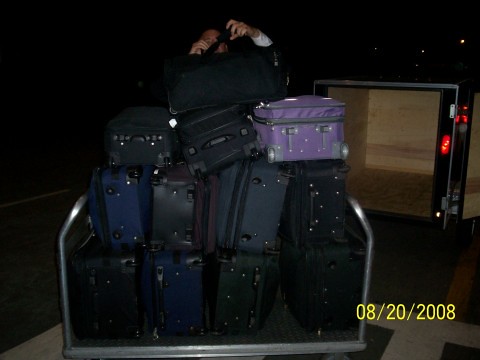The photograph, time-stamped 08-20-2008 in the lower right corner, captures an outdoor night scene at what appears to be an airport. Dominating the image is a large silver metal luggage cart with chrome sides, stacked high with approximately 12 pieces of luggage in varying colors, including black, navy blue, gray, dark purple, and medium purple. The cart, lacking a rear gate, holds suitcases layered in a meticulous arrangement—four on the bottom, four atop those, three on the next level, and finally one standing upright.

A man, only partially visible, is seen stacking a suitcase on top of the pile. He is wearing a dark suit with a white shirt visible at the sleeve, appearing Caucasian, with his head and hands just peeking above the luggage. On the right side of the photograph, an open trailer, shrouded in darkness, suggests he might be loading or unloading the suitcases. The background is predominantly dark, punctuated only by the red brake lights of a vehicle, highlighting the nighttime setting.